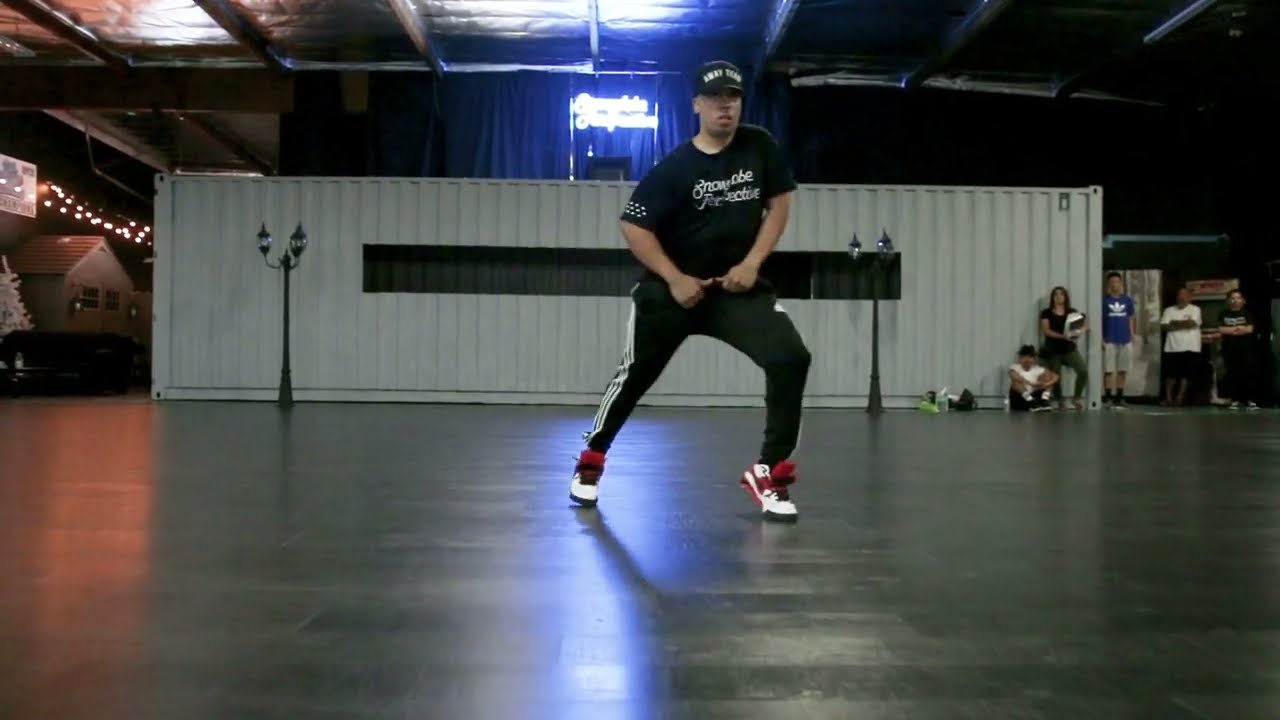In the image, a man is captured mid-dance in a large indoor room with a concrete floor. The space features raw insulation and lattice or boards visible in the ceiling, adorned with vibrant neon lights. The man, positioned centrally, is wearing a black cap with white lettering, a black t-shirt adorned with white lettering in the center and white dots on the sleeves, and black track pants with white stripes running up the sides. His sneakers are white with red and black accents. Striking a dynamic, somewhat unconventional dance pose, he has one leg lunged forward and the other set back with his hands positioned by his waistband, and his body leaning to one side. 

In the background, along the room's edge, several people stand in a line, watching him. Mostly cross-armed, they seem intrigued by his movements. To the left, a white Christmas tree and some house-like props are visible, adding to the eclectic decor. Behind the man, a white wall with a long window cut-out stands, flanked by streetlamp posts emitting a blue glow. This striking blend of elements sets a unique scene that enhances the focus on the solitary dancer.